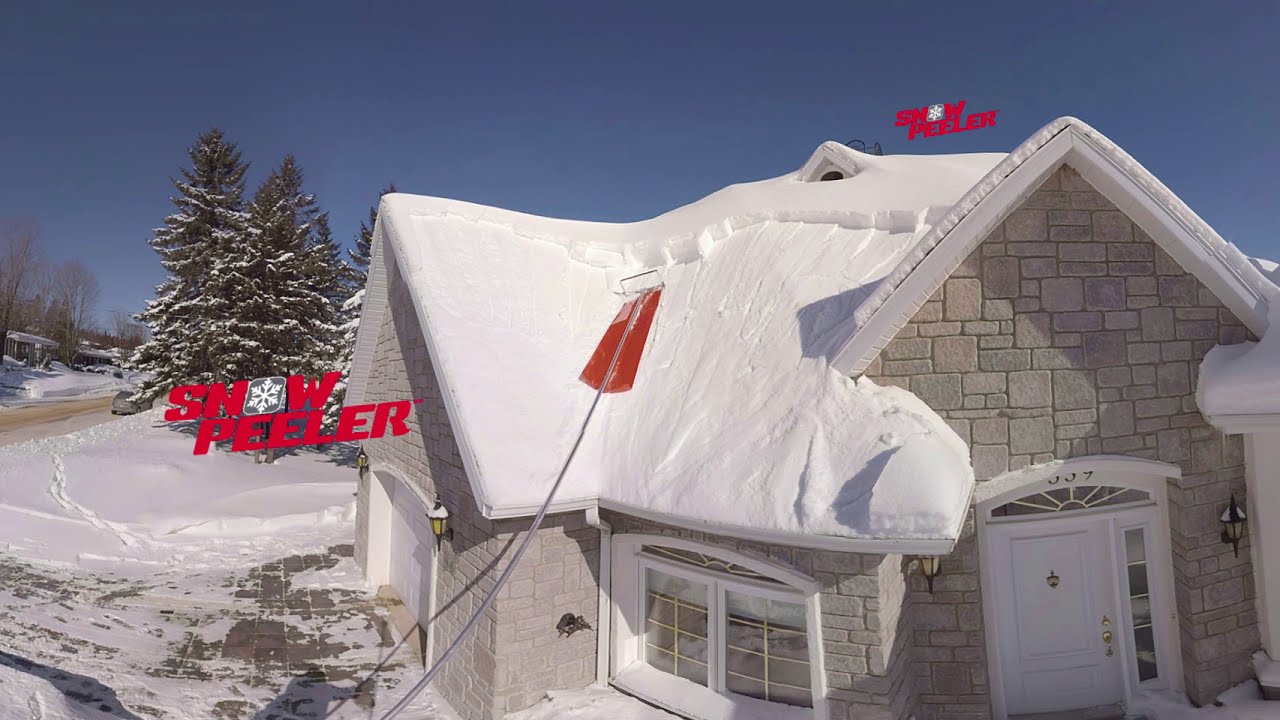Amid a serene winter wonderland, a quaint, tan-colored brick house is cozily nestled under a thick blanket of snow. This idyllic scene captures the essence of a snowy, suburban haven. The house features a welcoming doorway, several windows, and a garage to the left. Surrounding the home are towering evergreen trees, reminiscent of classic Christmas imagery, standing tall against the snow-covered ground.

The sky above is a strikingly clear, deep blue with a hint of purple, casting a serene brightness over the landscape despite the high accumulation of snow. Against this peaceful backdrop, a unique red "snow peeler" device stands out, mounted on the roof. The bright red text above the roof clearly reads "Snow Peeler," indicating the tool's purpose. The snow peeler, with its long, metal rod and a flipper-like end, is designed to remove heavy layers of snow from rooftops, ensuring the house remains safe and accessible during winter. It’s a functional touch to an otherwise picturesque, snowy suburban scene.